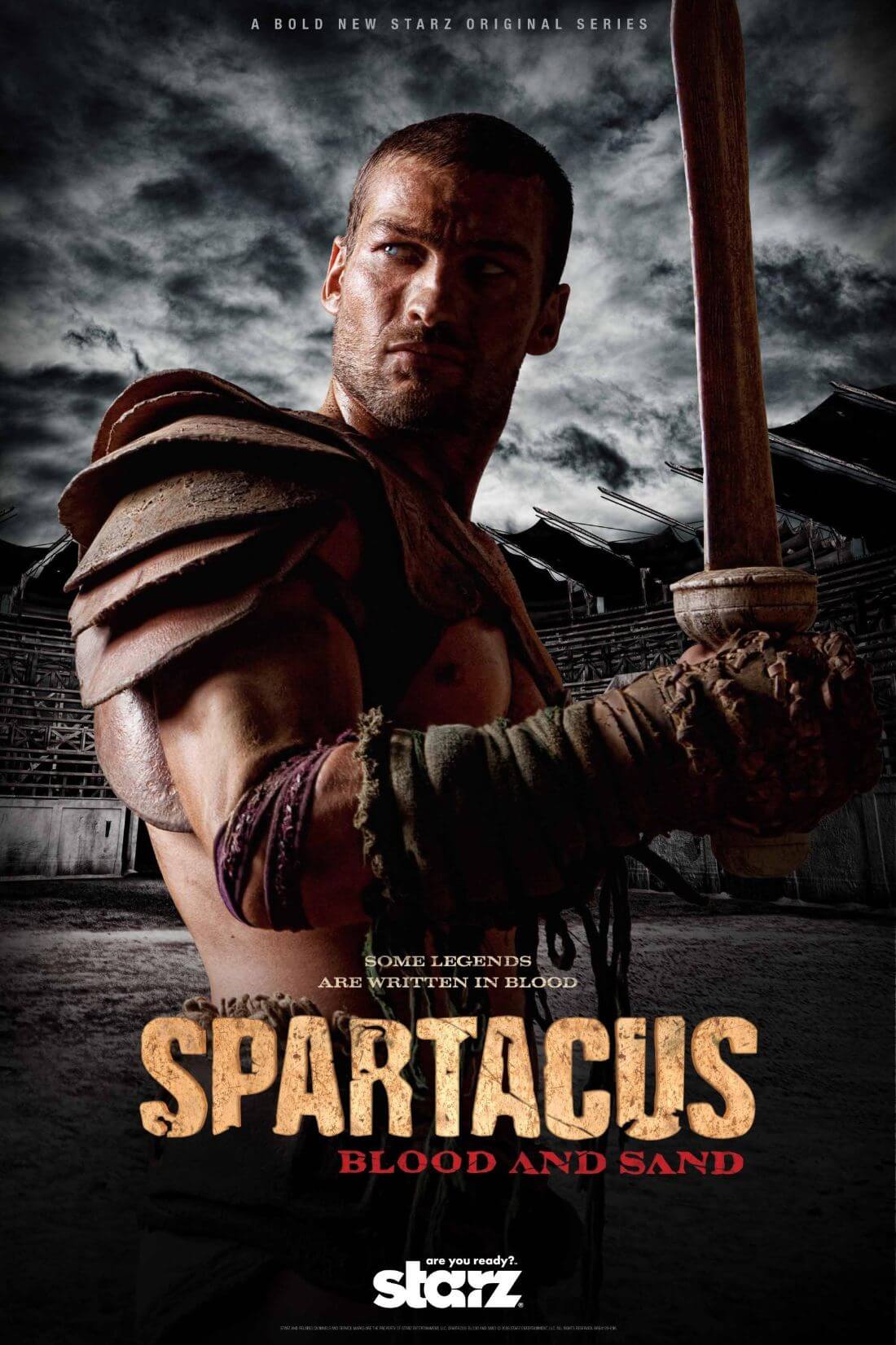This detailed promotional poster for the television series "Spartacus: Blood and Sand," a bold new Stars original series, prominently features the gladiator Spartacus. At the very top, in small white letters, it declares, "A bold new Stars original series." Dominating the center of the poster, Spartacus is depicted in a powerful side profile. He stands with his right arm bent at the elbow, holding a sword pointed toward the sky. His attire includes several leather shoulder pads (epaulets) and leather and cloth wrappings around his right hand, wrist, and forearm. His muscular frame is partially visible, with the image cutting off around his hips. The background is a stark black and white depiction of an ancient arena, suggesting spectator stands amidst a dark, cloudy sky. Centered at the bottom of the poster, the tagline "Some legends are written in blood" is inscribed in white text. Below this, in bold yellow letters, is the title "Spartacus," followed by "Blood and Sand" in red text, slightly offset to the right. Finally, the Stars logo is featured at the bottom of the poster, confirming this gripping new series.